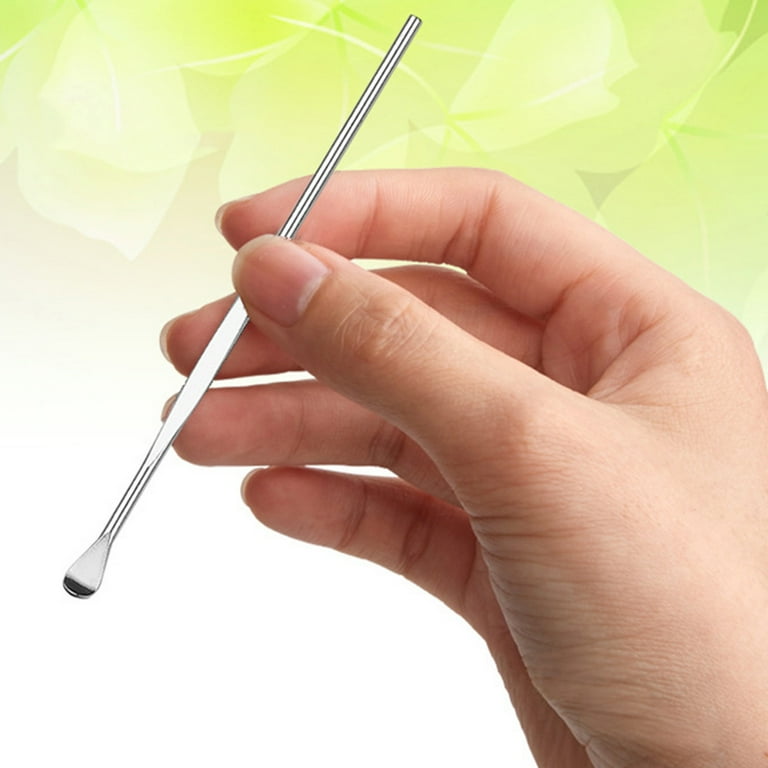The detailed close-up photograph captures a right hand, Caucasian, holding a slender, metal tool that appears silvery-white. The fingers are positioned towards the left side of the image, gripping the instrument, which flaunts a slight curvature at its flattened, spoon-like tip. This tool could be used for ear cleaning, scraping, or even carving intricate details, given its refined and delicate end. The background, though varied, reveals a predominantly white lower section and a blurred green, leaf-like abstract pattern above. The overall setting provides a clear focus on the metal tool, ensuring its features are highlighted against the indistinct backdrop.